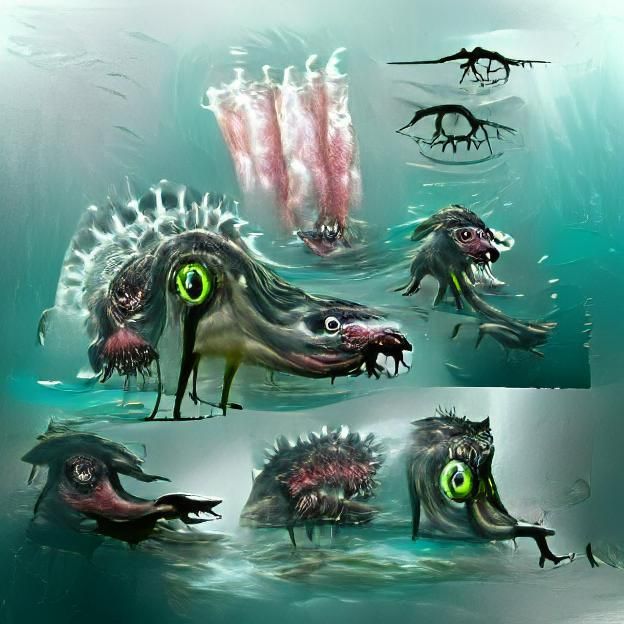In this detailed underwater-styled painting or drawing, primarily rendered in a teal or blue-green color, the artist depicts a vertical rectangular scene populated by a series of custom-made creatures. Dominating the image is a repeating central character, a lizard or alligator monster-like entity with a long face, rounded snout, and big, multicolored eyes—dark green, light green, and black. This entity's head, sometimes adorned with a green hat or white spikes, appears multiple times, presenting subtle variations.

Set against a futuristic and surreal background featuring shades of gray, purple, and white, and occasionally intersected by pink strips of paint, the scene presents an imaginative underwater realm. In the top section of the image, there is a depiction of a bizarre, sludge-like monster with a green eye on the side, another googly eye at the front, and a stringy red, bloody mouth. The middle part of the image showcases two squid-like creatures and a red-and-white entity. In addition, black silhouettes resembling dragons and AI-like fish enhance the fantastical quality of the scene.

The bottom part of the image features three more horrifying creatures, each with unique and menacing features, including another one with a green eye. The entire composition, lacking any text, appears as a modern art piece or something inspired by video game aesthetics, suggesting an AI-generated creation. The overall effect is that of an intricate, highly detailed, and otherworldly underwater tableau.